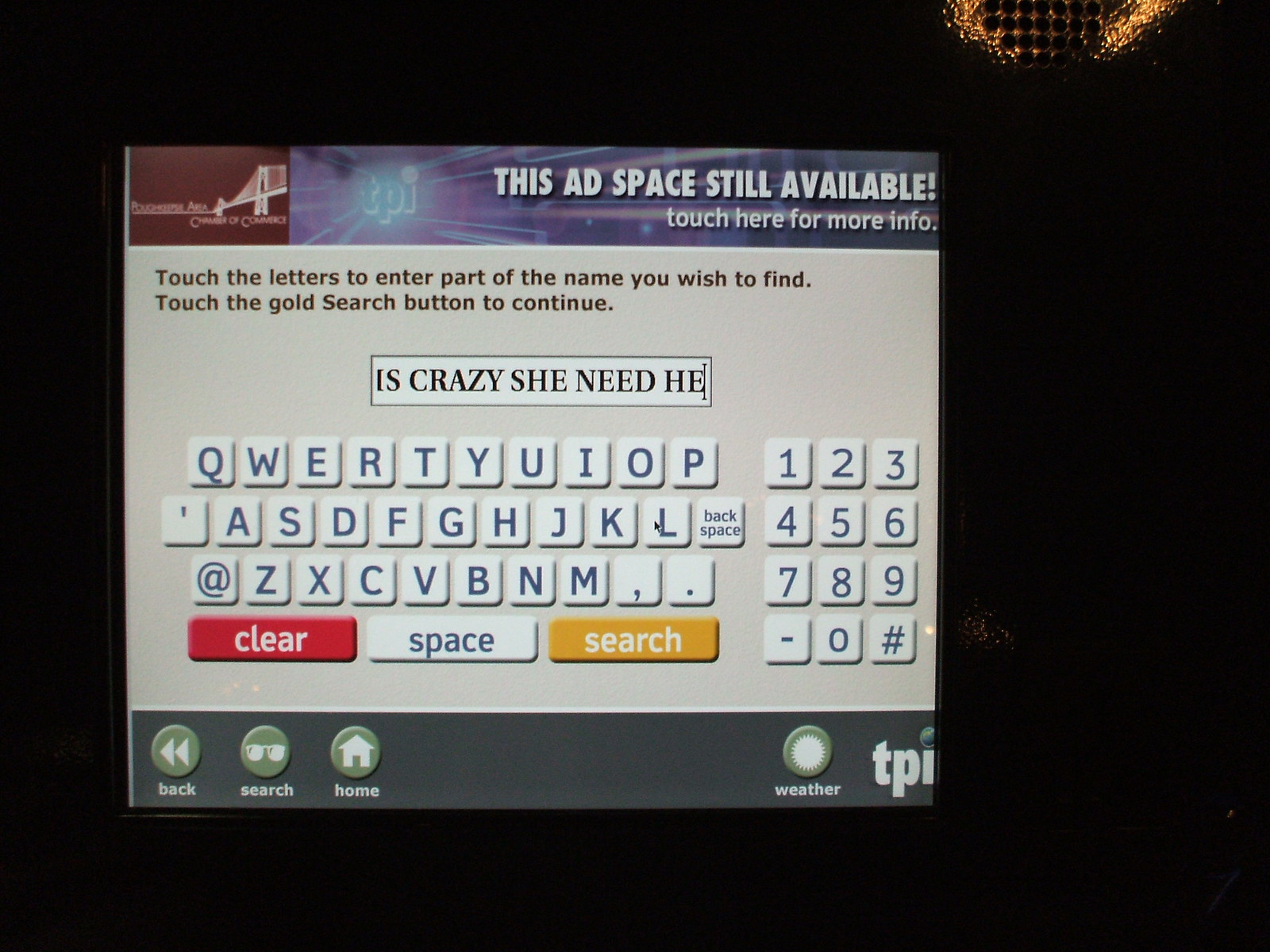The image features a central rectangular digital screen set against a dark background, possibly inside a dark room. The screen displays a virtual QWERTY keyboard with letters and numbers, 1 through 0, situated on the right side, alongside symbols like a dash and pound sign. Text instructions are visible at the top of the screen, stating, "Touch the letters to enter part of the name you wish to find, touch the gold search button to continue." At the very top, there's a banner saying, "This ad space still available, touch here for more info," next to a white and brown drawing of a bridge. The bottom of the screen hosts functional buttons for back, search, home, and weather. Above these buttons, a typed message reads, "is crazy, she need help," with an arrow indicating the letter 'L', suggesting a possible keyboard input error. The screen's layout suggests it could be part of an interactive system, perhaps a touch screen for data entry, commonly found in a service setting like a bank.